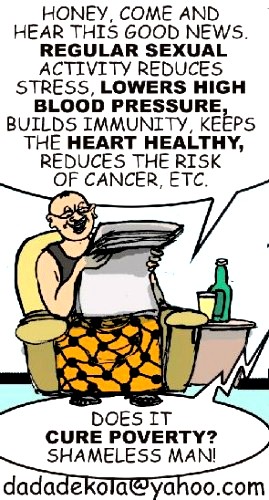In this cartoon-style comic strip, a man is depicted sitting comfortably on a yellow chair, dressed in orange pants and a black shirt, with a newspaper in hand. He also seems to have a blanket with little dots draped over his lap. He wears glasses and has minimal hair. Beside the man, a green bottle and a glass with yellow liquid rest on a side table. A text bubble above him reads, "Honey, come here, this is good news. Regular sexual activity reduces stress, lowers high blood pressure, builds immunity, keeps the heart healthy, reduces the risk of cancer, etc." In response, a voice off-panel, presumably his wife, jokingly retorts, "Does it cure poverty, shameless man?" Below the comic, the email address dadadacola@yahoo.com is provided, possibly indicating the source of the comic.